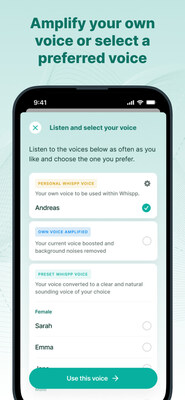**Descriptive Caption**

The image portrays a detailed mock-up of a smartphone screenshot. The background is a light teal color interspersed with horizontal bands of white. At the top, within a dark teal banner, the text reads, "Amplify your own voice or select a preferred voice." The device has a dark black bezel with the time "941" displayed in bold white text at the top, indicating military time. To the right, icons show full cell phone signal, full Wi-Fi signal, and a fully charged battery.

Beneath this, a light teal section features a white circle containing a teal 'X,' sitting next to bold teal text that reads, "Listen and select your voice." Below this instructional header, black text states, "Listen to the voices below as often as you like, and choose the one you prefer."

A white rectangle follows with an adjacent brown-bordered rectangle, though the text within it is blurred and only partially readable as, "Personal... voice." Below, in black, it reads, "Your own voice to be used within WHIS APP." A dark gray gear icon appears beside this text, suggesting settings or adjustments.

The next section contains selectable voice options. "Andreas," highlighted in dark gray text with a teal circle and white check mark beside it, indicates a selected option. Another option within a light blue rectangle is labeled in bold blue as, "Own Voice Amplified," with a white circle (unchecked) on the right. It explains in black text, "Your current voice boosted and background noise removed."

Further down, another option with a dark teal border and lighter teal interior is titled "Present WHIS APP Voice" in dark teal text. This is explained in black text as, "Your voice converted to the clear and natural-sounding voice of your choice." Bold teal text label options for female voices are also listed: "Sarah," with a non-selected white circle, and "Ella," also non-selected.

Finally, at the bottom, a dark teal, oval clickable button with bold white text reads, "Use this voice," accompanied by a white arrow pointing to the right.